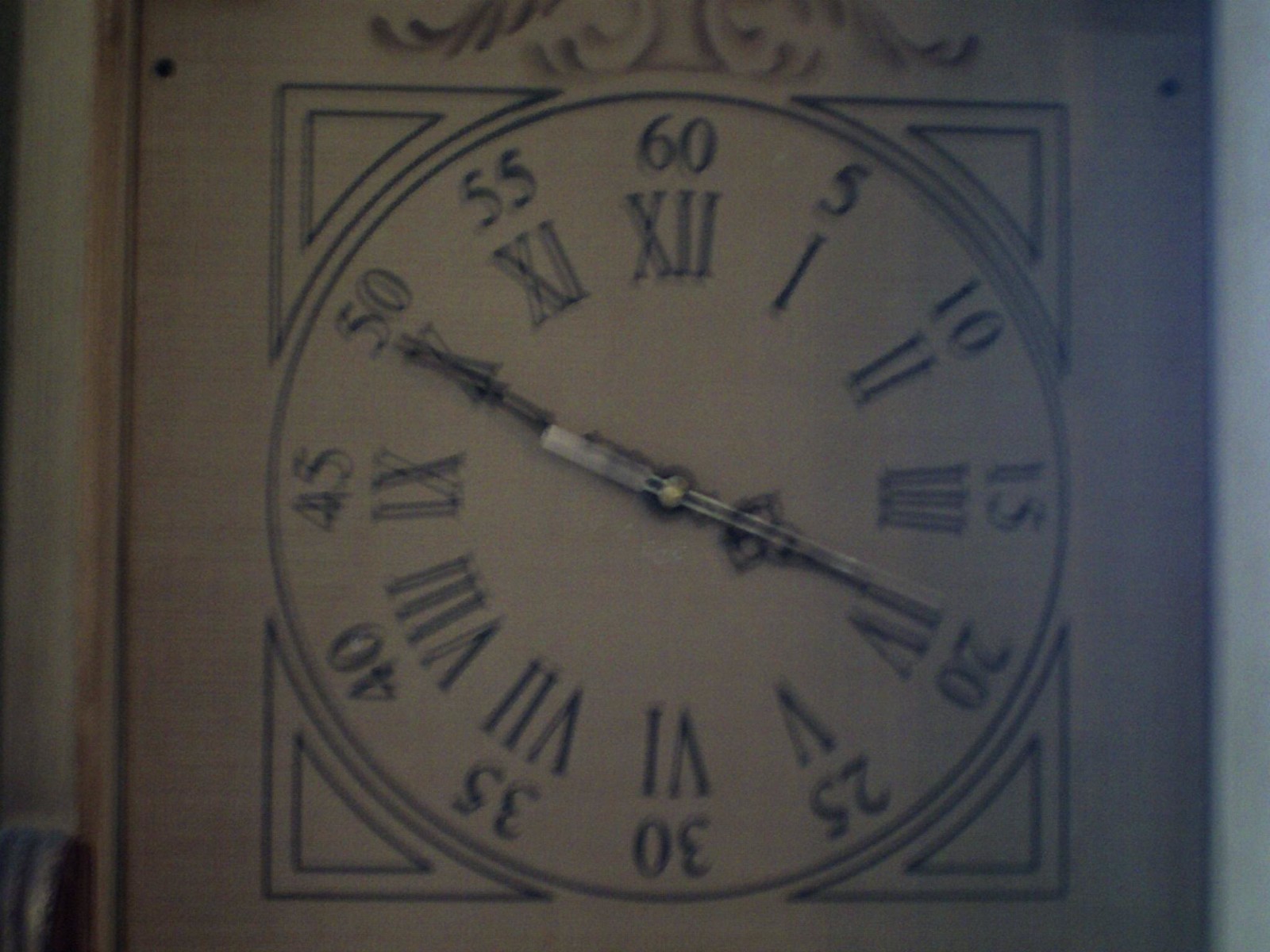This is a grainy, black-and-white close-up photograph of an ornate wall-mounted clock face with a black frame featuring rounded triangular designs at each corner. The clock face is set against what seems to be a backdrop of raw, exposed wood. It showcases both Roman numerals and regular numbers with dark blue Roman numerals marking the hours from III to XII and regular minute markers in five-minute increments from 5 to 60 encircling the clock. Notably, the time reads around 10:19 or 10:20. The clock's hands are intricate, with black metal designs for the hour and minute hands and a thin silver second hand. Additionally, there is a decorative flourish resembling a leaf pattern above the clock face, contributing to the elaborate design. The overall image quality is quite poor, characterized by a blurry and low-light appearance.